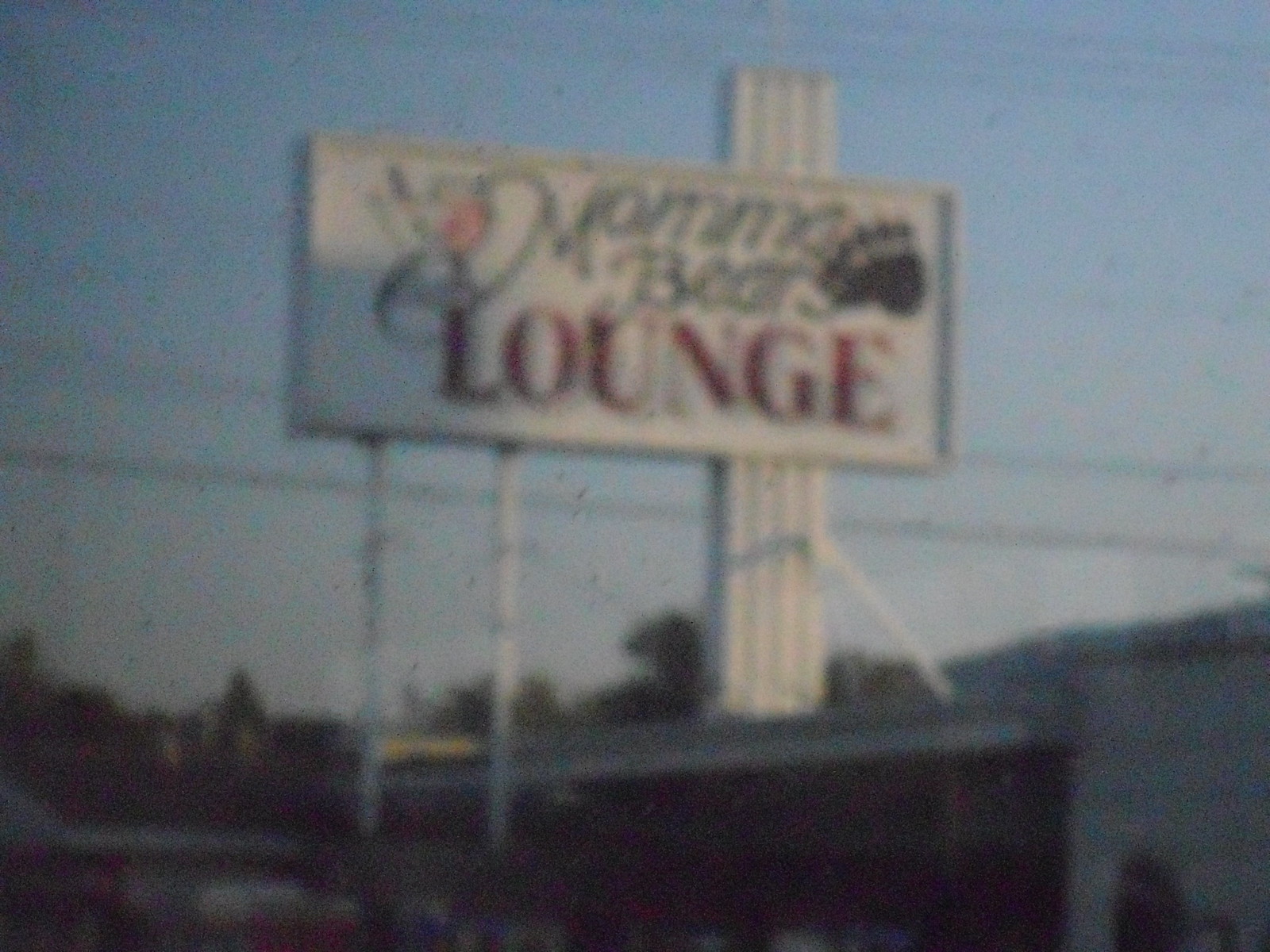The image is an extremely blurry and grainy photograph, likely taken decades ago, with dull colors characteristic of a vintage 35mm camera. The photo features a blue sky with a few scattered clouds, and a tree line is visible at the bottom. Dominating the foreground is a rectangular white sign attached to a building. The sign reads "Mama Bear Lounge" in green and red text, with a bear paw print in the upper right corner. The top part of the sign, listing "Mama Bear" in green cursive, is connected to three small white pipes and rests on a set of vertical white boards. Below, "Lounge" is written in bold red letters. The sign is mounted close to some electrical lines and appears to be supported by white legs resting against a chimney-like structure. Shadows of people can be seen in the vicinity, but they are not clearly visible. A closer inspection reveals what might be a martini glass on the left side of the sign, although the poor quality of the image makes it difficult to confirm. The overall ambiance suggests it could be a bar, possibly attached to a hotel or motel.